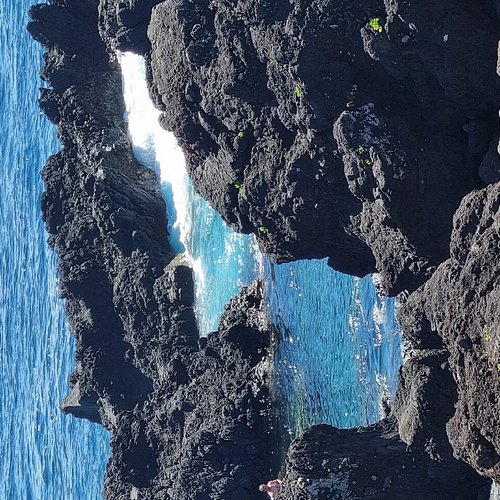This image, viewed at a 90-degree counterclockwise rotation, captures a rugged shoreline dominated by large, dark gray and charcoal-black rocks, possibly volcanic. The rocks, some casting shadows under the sunlight, form a prominent hollowed-out area, filled with bright blue ocean water, creating a striking contrast. Small patches of grass or weeds can be seen sporadically growing amongst these rocks. In the background, the expansive ocean showcases a calmer, lighter blue hue with horizontal wavy patterns and scattered white streaks of waves. This daylight photo exquisitely captures the interplay between the rough, textured rocks and the tranquil yet vivid blue ocean.